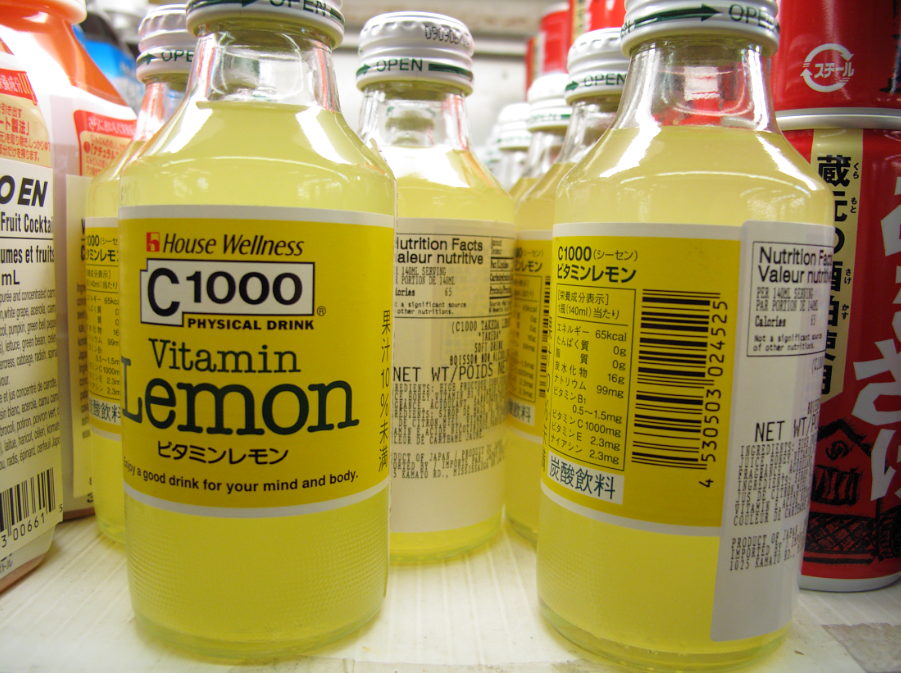The image captures an up-close view of a store shelf, refrigerator, or pantry, featuring three distinct products. Dominating the center, there are approximately seven bottles of House Wellness C-1000 Vitamin Lemon Drink, characterized by their light yellow hue. The labels prominently display the product name along with nutritional information. To the left, partially visible, is an unidentified container with the text 'fruit cocktail' on it. On the right side of the image, there are red cans of an unknown product or beverage neatly stacked two-high.